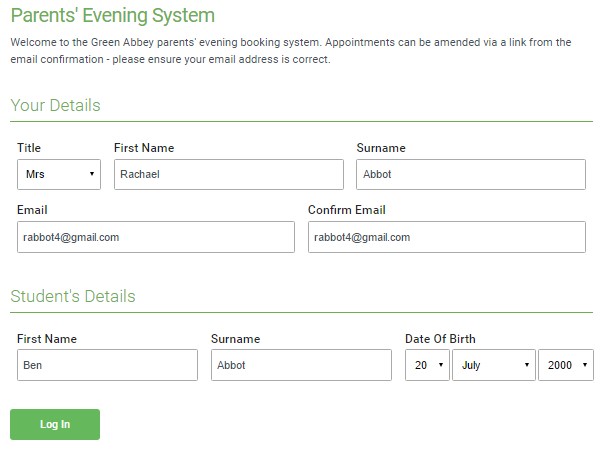**Welcome to Green Abbey Parents Evening Booking System**

This is the official webpage for the Green Abbey Parents Evening Booking System. Here, you can book and manage appointments for the upcoming parents' evening. Below is a detailed walkthrough of the form presented on the page:

1. **Introduction Text**
   - "Welcome to Green Abbey Parents Evening Booking System. Appointments can be amended via a link from the email confirmation. Please ensure your email address is correct."

2. **Personal Details Section**
   - **Title**: A dropdown menu with pre-selected option "Mrs."
   - **First Name**: The text box contains "Rachel".
   - **Surname**: The text box contains "Abbott" (with one "T").

3. **Contact Information Section**
   - **Email**: The text box contains "Rabot4@gmail.com".
   - **Confirm Email**: The text box, again, contains "Rabot4@gmail.com".

4. **Student Details Section**
   - **Student's First Name**: The text box contains "Ben".
   - **Student's Surname**: The text box contains "Abbott" (spelled as A-B-B-O-1-T in the voice description, corrected to A-B-B-O-T-T).
   - **Date of Birth**: 
     - **Day**: A dropdown menu with "20".
     - **Month**: A dropdown menu with "July".
     - **Year**: A dropdown menu with "2000".

5. **Login Button**
   - There is a green "Login" button located at the bottom for submitting the entered details.

In summary, the webpage provides a user-friendly interface for parents to book, review, and manage appointments for parents' evening by entering their and their child's details, along with a prominent login button for easy access.